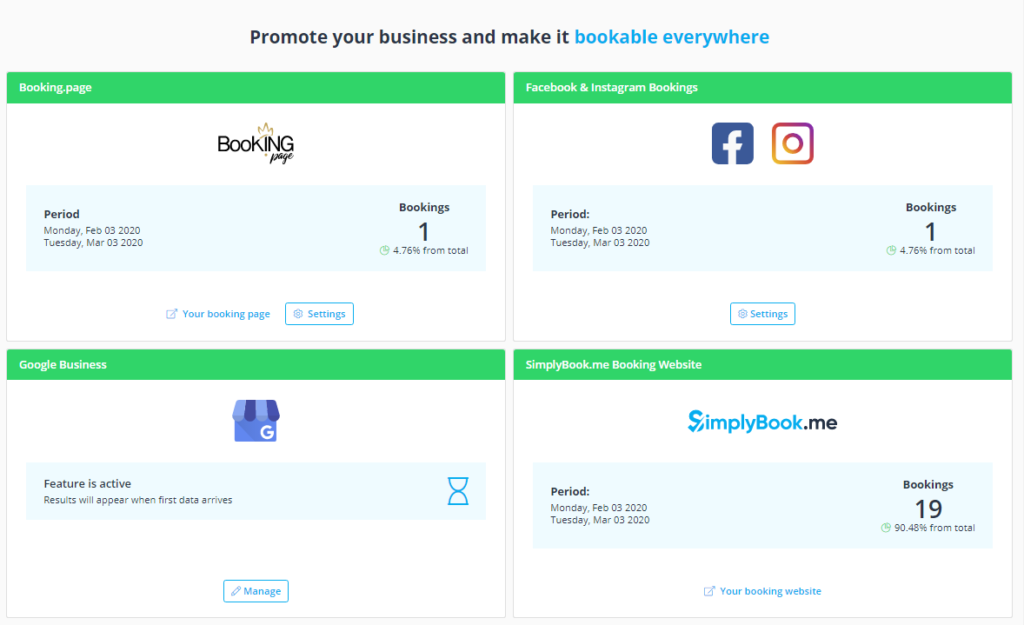The image, sourced from a website, is set against a white backdrop and consists of four smaller images arranged in two columns. The first column contains two images stacked vertically on the left, mirrored by two similarly arranged images on the right.

At the top center of the page, the text reads "Promote your business and make it" in black, followed by "bookable everywhere" in blue.

**Top Left Image:**
- **Backdrop:** White.
- **Top Bar:** Green with "Booking Page" in white text on the left.
- **Center Text:** "Booking Page" with a small gold flower above the word "Booking."
- **Blue Bar:**
  - Left: "Period"
  - Below: "Monday Feb 03-2020" and "Tuesday March 03-2020"
  - Right: "Bookings"
  - Below: Numbers “1”, “4”, “7”, “6”, “9”, “6” from total.
  - Blue text: "Your Booking Page"
- **Bottom Right:** Blue outlined circle with the word "Settings" in blue.

**Top Right Image:**
- **Top Bar:** Green with "Facebook & Instagram Bookings" in white text.
- **Center:** Blue box with a white lowercase "f" for Facebook and a camera icon for Instagram.
- **Blue Bar:**
  - Left: "Period:"
  - Below: "Monday Feb 03-2020" and "Tuesday March 03-2020"
  - Right: "Bookings"
  - Below: Numbers “1”, “4”, “7”, “6”, “9”, “6” from total.
  - Center: Box with gear icon and "Settings" to the right in blue.

**Bottom Left Image:**
- **Top Bar:** Green with "Google Business" in white text.
- **Center:** Blue tent-like shape resembling a shop awning with a white "G" in the bottom right.
- **Blue Bar:**
  - Left: "Feature is active. Results will appear when first data arrives."
  - Right: Blue outline of an hourglass.
  - Center: White box outlined in blue with a pencil icon on the left and "Manage" in blue text.

**Bottom Right Image:**
- **Top Bar:** Green with "SimplyBook.me Booking Website" in white text.
- **Logo:** "SimplyBook" in blue, followed by ".me" in black.
- **Blue Bar:**
  - Left: "Period:"
  - Below: "Monday Feb 03-2020" and "Tuesday March 03-2020"
  - Right: "Bookings" in black
  - Below: Number “19”, percentage “90.48%” from total.
  - Center: White box with a blue arrow in the top right and "Your Booking Website" in blue.